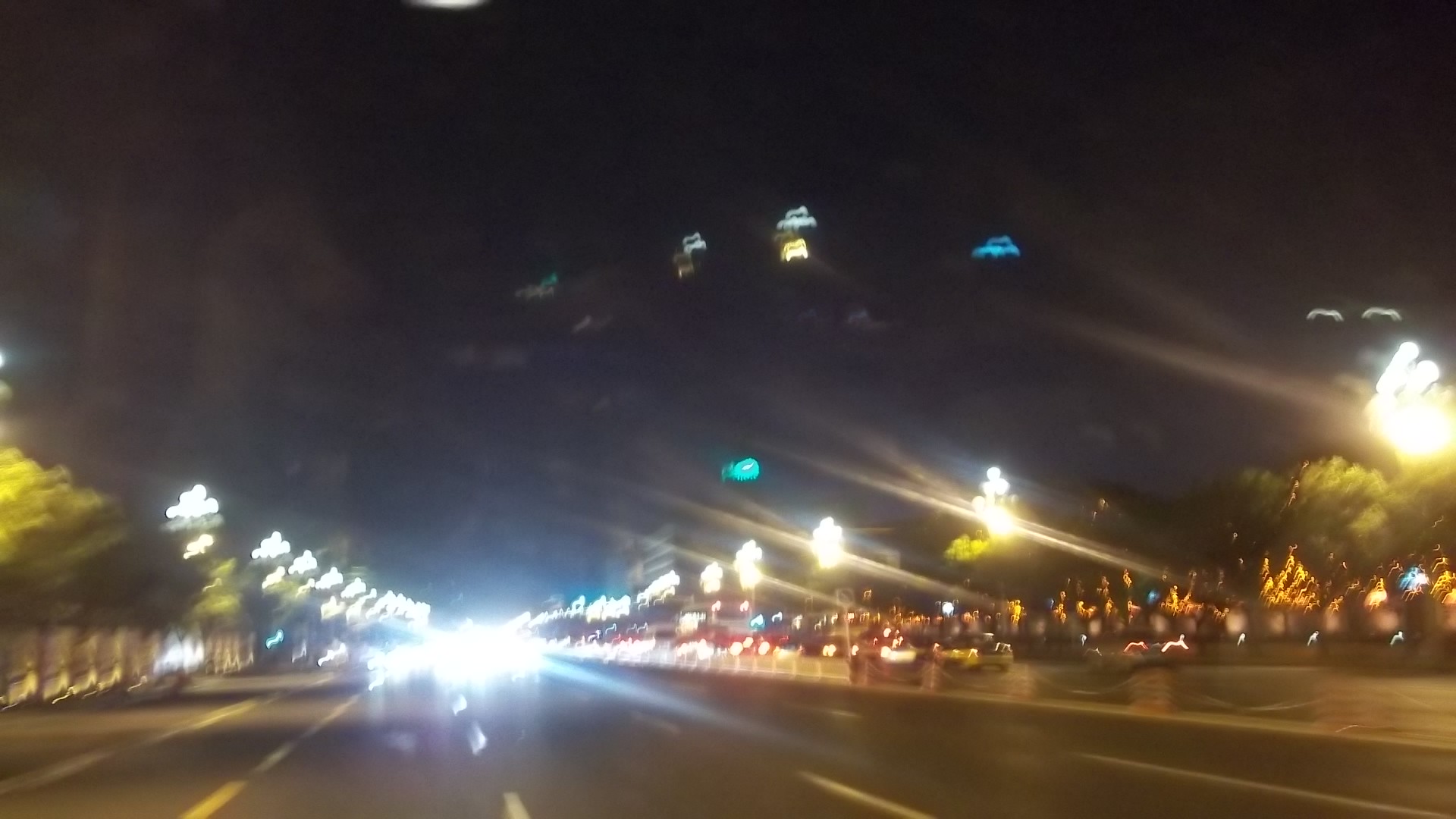This nighttime photograph captures a blurry view of a roadway as seen from the rear window of a moving vehicle. Toward the bottom center of the image, the lights of approaching cars create a streaked effect, hinting at the motion of the vehicle and the late-hour setting. To the right side of the frame, a separate roadway branches off in a different direction, populated by additional vehicles whose headlights also appear blurred. A median strip divides these two roadways, adding structure to the chaotic array of moving lights. In the far right corner of the image, trees are faintly visible, shrouded in darkness. Above, LED lights from surrounding buildings punctuate the skyline, adding an urban touch to the night scene.